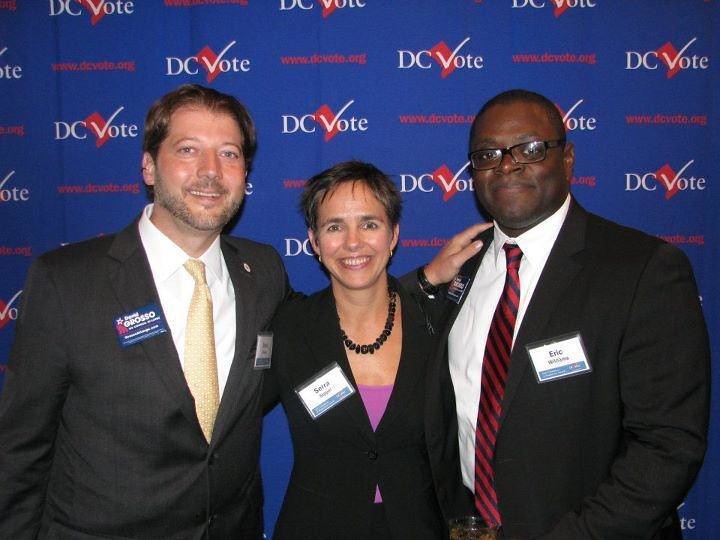In the photograph, three individuals are smiling and standing in front of a vibrant blue backdrop, which prominently features the logo for dcvote.org, with "DC" and a check mark forming the "V" in "vote" in white against a red background. 

The individual on the left is a white man with short brown hair and a five o'clock shadow, dressed in a dark gray to black suit with a white button-up shirt and a distinctive yellow tie. He wears a blue name tag with white text on the left side of his blazer, and his name is Daniel Grosso.

In the center stands a white woman named Sierra, with short black hair, adorned with a black stone necklace. She is dressed in a black blazer, which is buttoned up, partially covering a light purple blouse, paired with a white and blue name tag situated on the left side of her blazer. 

On the right is a black man named Eric, with short black hair and black-framed reading glasses. He is dressed in a black suit with a white button-up shirt and a tie featuring red and dark blue stripes. His name tag, which reads "Eric" in black, is located on the right side of his blazer.

All three individuals are smiling warmly at the camera, creating a positive and engaging scene at what appears to be a formal event or convention.